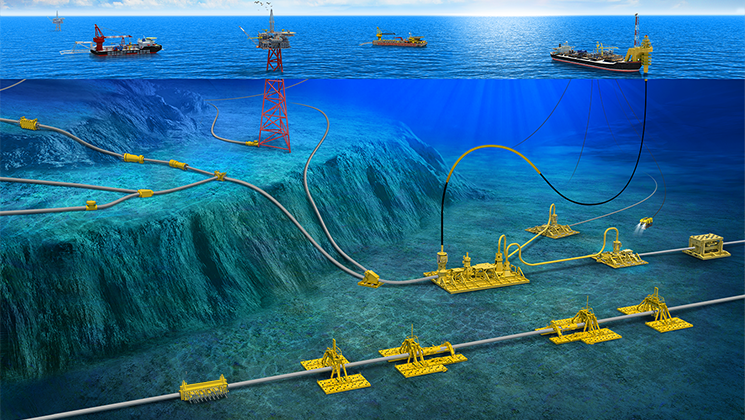The image showcases a captivating scene that simultaneously reveals both above and below the water surface of a vibrant, blue ocean. Above the water, we see three large boats, including one slightly larger and brown, bustling with people. To the side, a prominent metal framework stands on a small hill beside the water, with cables descending the hill into the ocean. 

Underwater, various contraptions appear to be fastened to the ocean floor, resembling railroads or long steel wires tethered by large yellow clamps. Each boat has extended lines or cables plunging into the depths, suggesting an operation where items are either being extracted from or deposited into the water. These underwater cables create a web-like formation connecting the boats to the seabed's metallic structures, adding an intricate layer to the scene. The rich blue hues of the ocean and sky enhance the overall serene yet industrial ambiance of this marine tableau.